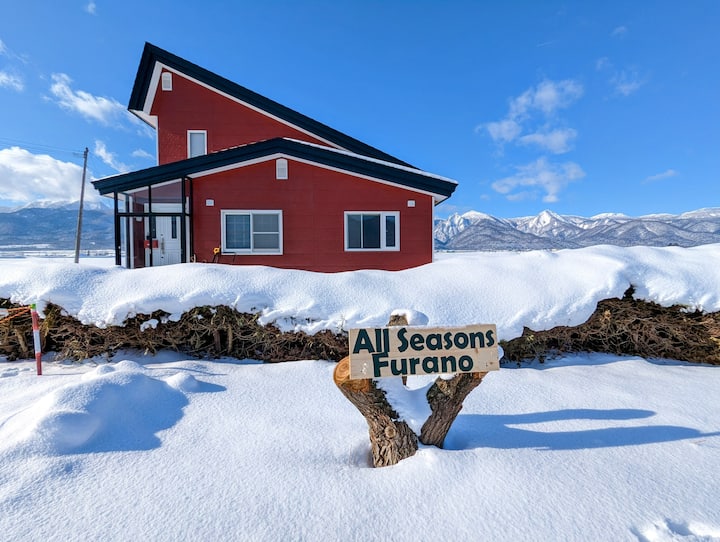In this picturesque daytime photograph, a solitary red cabin stands prominently in a snow-covered field under a deep blue sky scattered with white clouds. The cabin, with its striking red siding and contrasting white trim around the roof and windows, has a distinctive architectural style featuring a gabled roof on the first story and a uniquely angled roof on the second story, resembling a sideways number seven. To the left of the front, which showcases two windows, there is a glass-enclosed entryway outlined in white that leads into the main door. The roof sides are black, adding a modern touch to the rustic cabin design.

In the foreground, a sawed-off tree trunk supports a wooden sign with black lettering that reads "All Seasons Furano". This sign adds a welcoming touch to the remote yet serene setting. A hedge of snow-covered plants lines the snowfield, enhancing the wintry atmosphere. Power lines seen to the left subtly connect this idyllic scene to the broader world, indicating it isn't entirely isolated. Behind the cabin, a majestic range of snow-capped mountains stretches across the background, completing this tranquil and scenic winter landscape.